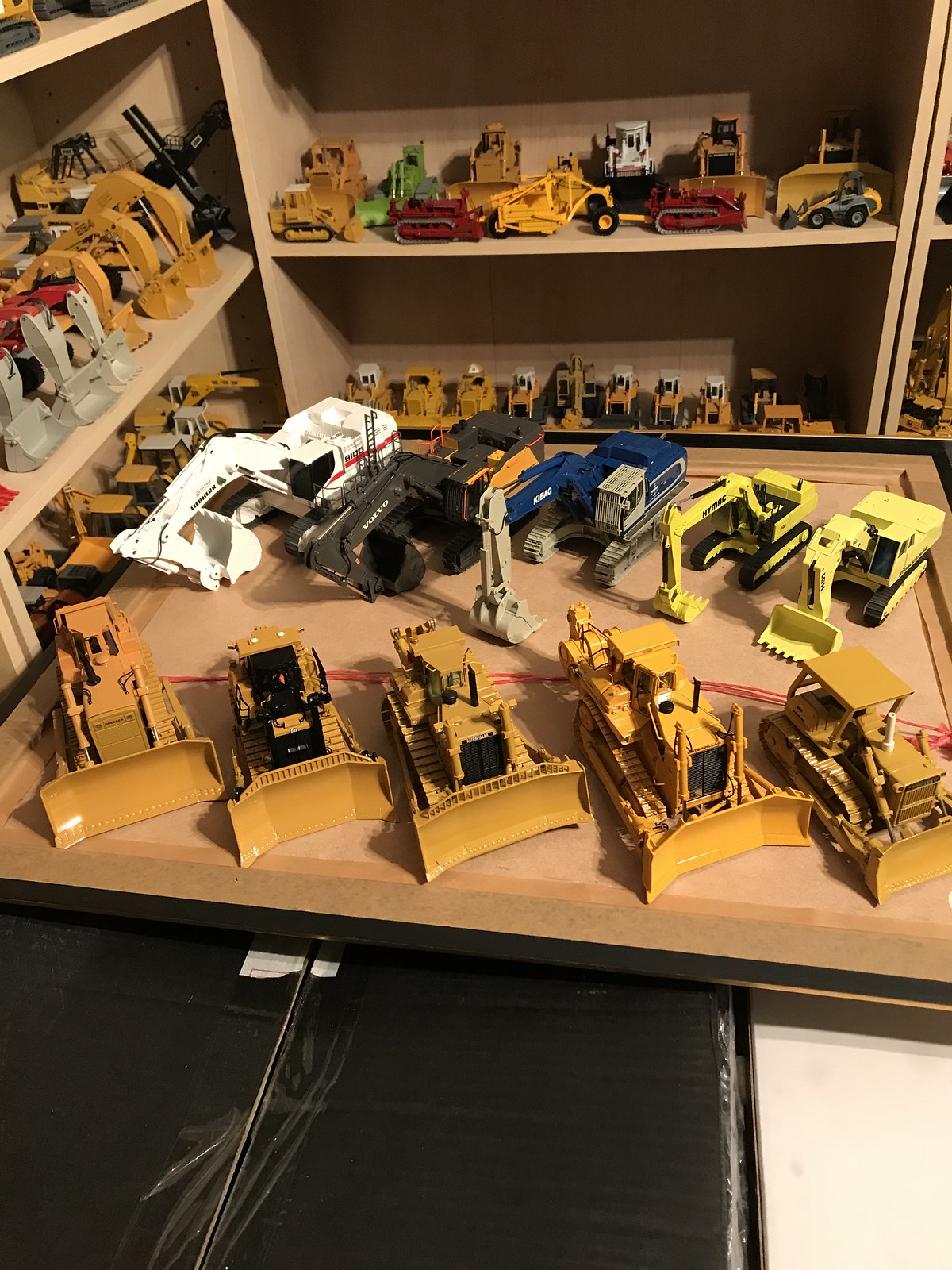In this detailed color photograph, we're presented with what appears to be a meticulously arranged collection of miniature construction vehicle models, likely in a boy’s room. The tabletop, seemingly made of an unfolded cardboard box placed atop additional cardboard boxes, displays an array of intricately designed models. The models in the front row are primarily yellow bulldozers, flanked by a variety of other construction machines such as yellow, blue with gray, entirely black, and white with red-striped excavators, one of which bears the “Volvo” brand. Surrounding the table on the back and left sides are light blonde wooden display units, each featuring two shelves brimming with more miniature construction vehicles. These shelves hold an extensive assortment, showcasing colorful models in brown, black, blue, yellow, white, red, and green hues, indicative of a passionate collector’s display. The room itself exudes a youthful charm, potentially a little boy’s sanctuary, reflecting a deep fascination with construction machinery.